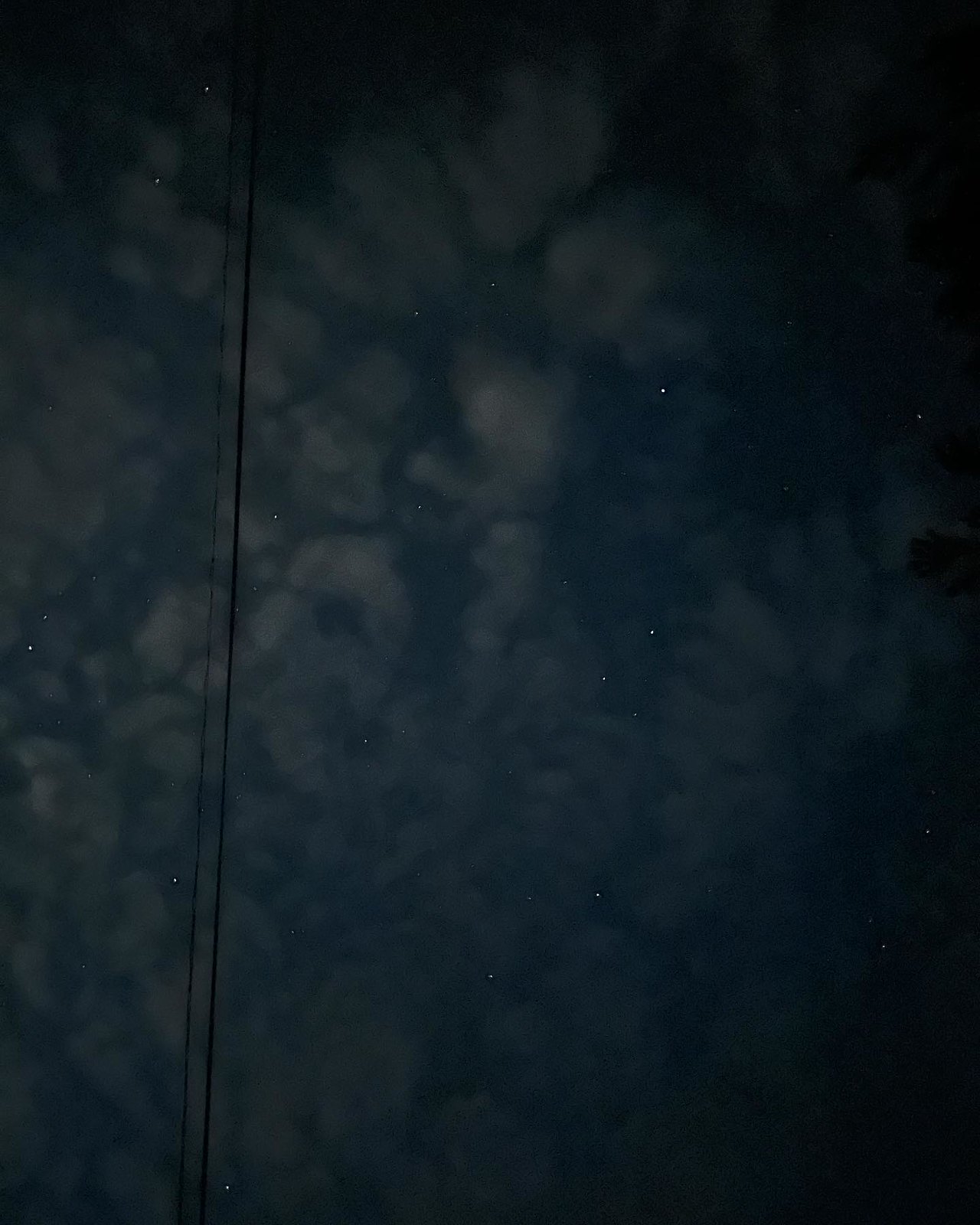The image presents a captivating view of the night sky, as if the camera is placed directly amidst the celestial expanse. It is nighttime, with the photograph exhibiting a subtle vignette effect, where the edges are engulfed in darkness, transitioning to a dark blue towards the center. Scattered across the sky are numerous tiny white dots, representing stars that, despite their size, appear remarkably bright. Draped across this star-studded backdrop are faint, wispy clouds, so translucent that the stars remain visible through their delicate veil. These clouds span much of the visible sky, adding a layer of ethereal beauty. On the leftmost part of the image, two vertical black lines, presumably power lines, ascend from the bottom left to the top left, grounding the celestial view with a touch of terrestrial reality.